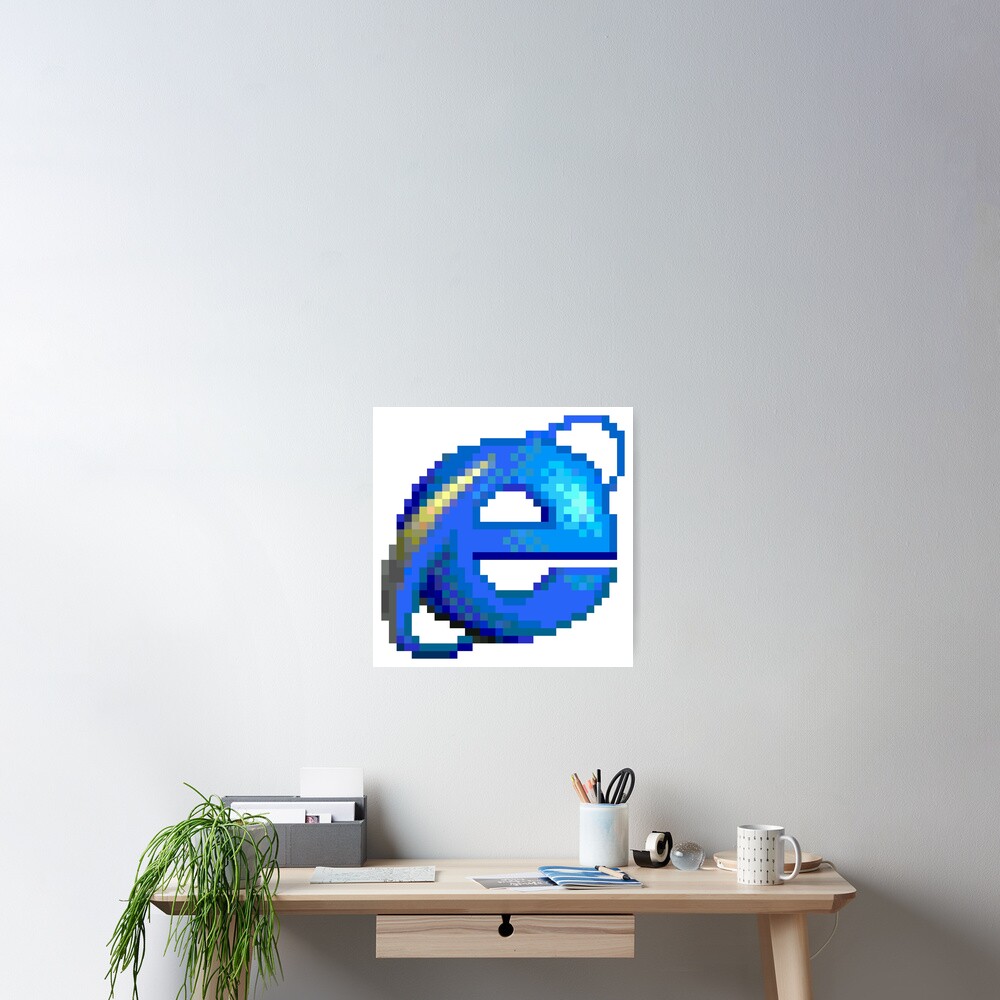In an office-like interior setting, a photograph captures a minimalist workspace against a slightly grayish-white wall. Dominating the background is a white square poster prominently displaying a pixelated Internet Explorer logo, characterized by a blue "E" with a gold ribbon-like swirl. Below this poster is a desk of pale brown wood, which includes a variety of organized items. To the left, a green plant cascades slightly over the edge. A gray document holder with scattered documents, including a noticeable blue booklet, sits towards the back. Central on the desk, a white cup holds several pencils and pens, next to a white mug with polka dots. A tape dispenser is situated nearby, along with a small white area lamp positioned to the right, arching at a 90-degree angle to illuminate the workspace. The neat arrangement of neutrals and focused elements like the plant and the iconic logo create a balanced, professional atmosphere.